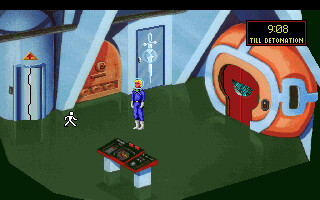The image is a screen capture from a video game set in a futuristic environment, viewed from a three-quarter perspective. The scene showcases a room with a green cement-like floor and gray walls on the left. Dominating the far right of the room is an oval orange structure with two central red double doors, which might function as an entryway. Just left of center, a small figure clad in a blue spacesuit is visible. The figure's suit features a black belt, silver gloves, silver boots, and a clear, globe-like helmet. To the far left, there appears to be a turbo lift or elevator door, which may have a medical symbol on it. Prominently closer to the foreground, left of center, stands a black control panel supported by two gray pedestals with various colored knobs, including red. In the upper right corner of the screen, there is a black rectangle with a red outline, displaying a timer set at "9:08" in yellow letters and the text "TILL DETONATION" below it, indicating a countdown to an impending event.